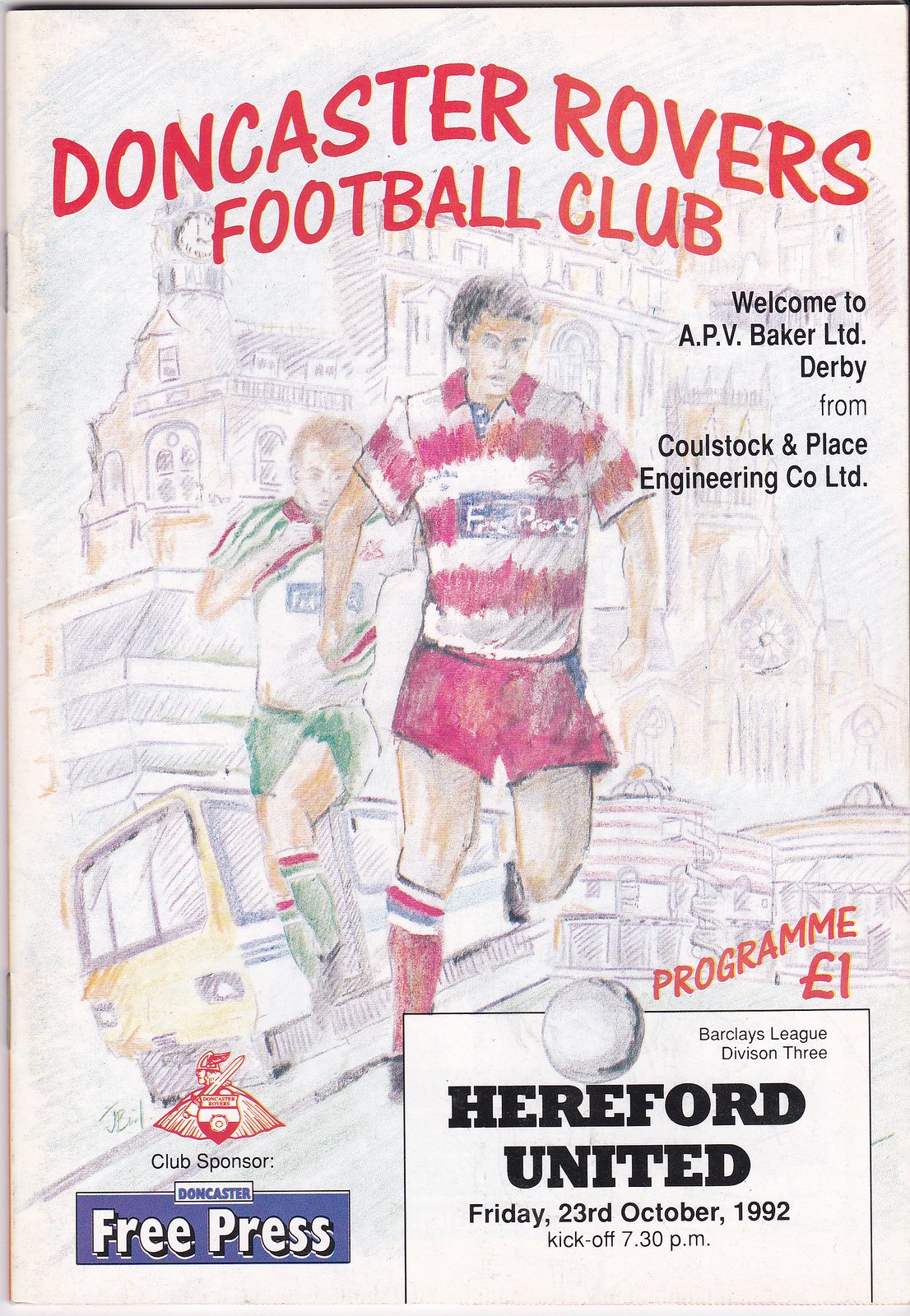The cover of this Doncaster Rovers Football Club program, priced at one Euro, features a detailed, colorful drawing of two men playing soccer. The man in the forefront is clad in a red and white striped uniform with red shorts, kicking a soccer ball, while behind him, another player in a white uniform with green shorts looks on. The background showcases muted-tone sketches of buildings and a bus or subway to the bottom left. Bold, handwritten-style red letters at the top announce "Doncaster Rovers Football Club" in an upward arc. The right side in black ink extends a welcome to APB Baker Limited Derby from Cool Stock and Place Engineering CO Limited. At the bottom, it states “Hereford United” in black, with the match date, “Friday 23rd October 1992,” kickoff time “7.30pm,” and league information, “Barclays League Division 3.” The iconic red Doncaster Rovers logo, depicting a Viking with a sword, is forthrightly displayed, and beneath it, in a blue box with white lettering, it reads "Free Press, Doncaster Free Press."